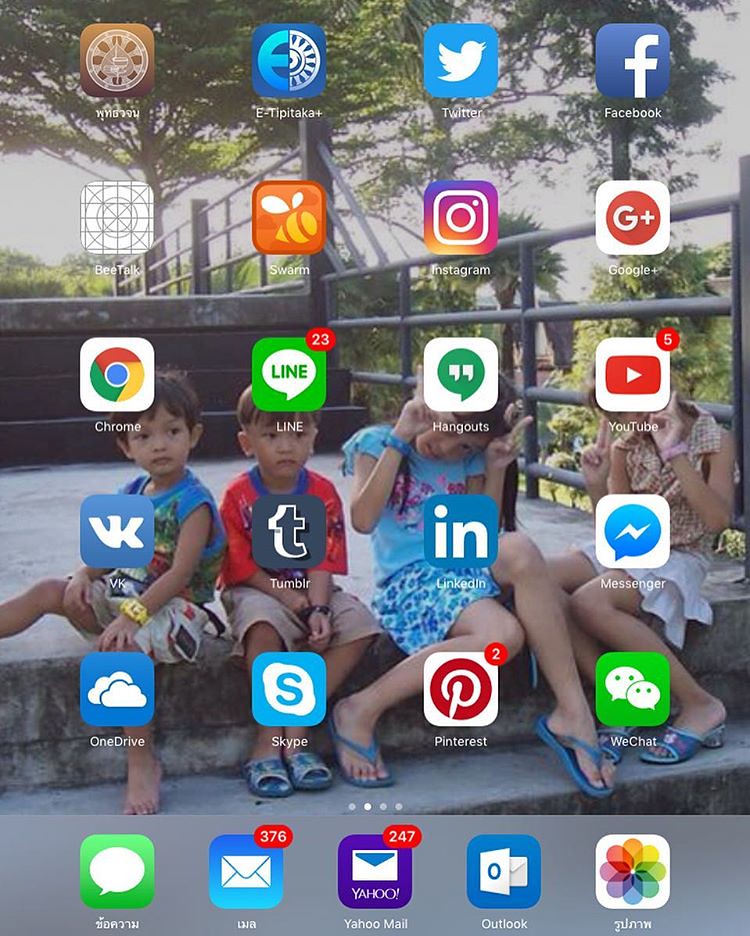This screenshot captures the home screen of a smartphone or an iPad, showcasing a variety of apps. At the top of the screen, a brown app icon with a white circle is present, followed by a blue app icon featuring a partial white circle and a letter 'E'. Below these, familiar apps like Twitter, Facebook, and one with an unreadable or broken icon, possibly labeled "Beetalk," are visible. The "Swarm" app, identifiable by its bee-themed icon, is next, alongside Instagram, Google+, Chrome, Line, Hangouts, YouTube, VK, Tumblr, LinkedIn, Messenger, OneDrive, Skype, Pinterest, and WeChat.

At the bottom of the screen, several apps appear with names displayed in a different language. These include the Messages app, Mail, Yahoo Mail, Outlook, and Photos. The background image features a scenic setting with four children—two boys and two girls—sitting on cement steps, surrounded by natural elements, a half wall, and a metal fence. The detailed arrangement and visual elements provide a glimpse into the device owner's diverse app usage and their cherished background photograph.